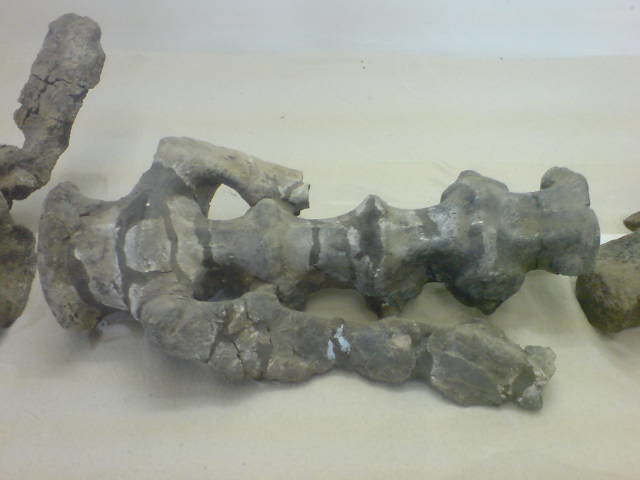The photograph, in landscape orientation, showcases a gray, petrified skeletal structure, possibly a spinal cord, that appears to be made of stone or charred bone. Central to the image, the structure is laid on its side on what seems to be a white table or light cream paper surface. The central piece features a series of vertebrae-like segments extending vertically, with smaller horizontal intersections. Additional fragments of the structure are positioned to the left and right, partially out of frame. The background features a soft blue hue that contrasts subtly with the lighter foreground, indicating an indoor setting, likely a museum. The detailed and realistic style of the photograph accentuates the relic's textures and layered composition, underscoring its significance as a preserved artifact.